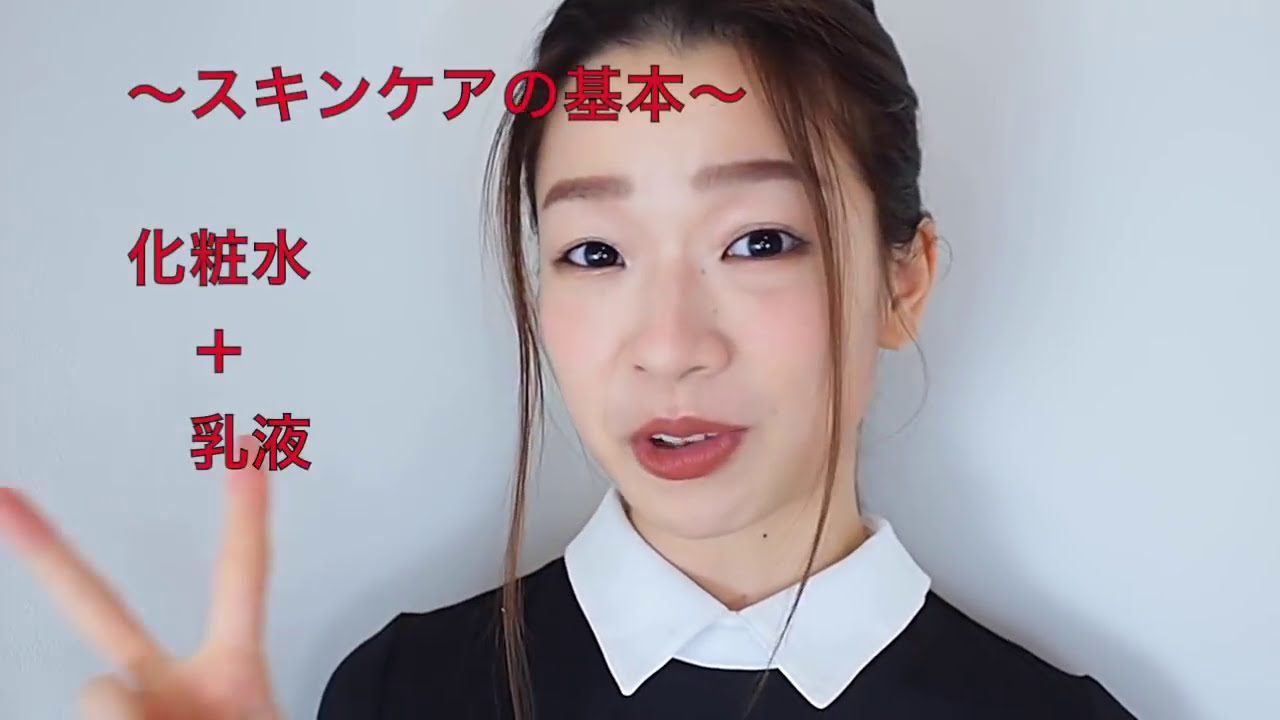The image depicts a young Asian woman standing in front of a light gray drywall background. She is dressed in a dark-colored sweater with a crisp white collar buttoned all the way up, creating a sharp contrast. Her dark hair is tied back, but two sections frame her face, extending down to her shoulders. She is holding up a peace sign with her right hand near the bottom left corner of the photo. Overlaid on the upper left-hand side of the image is red text featuring Asian characters, possibly Japanese or Chinese, with a distinct plus symbol in the middle. The woman’s appearance is marked by dark brown eyes, thick brown eyebrows, and red lips, adding to her youthful and vibrant look.